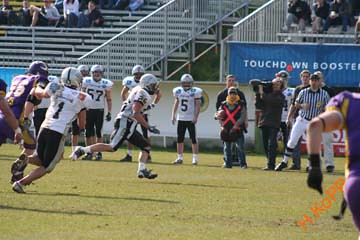This digital photograph captures an outdoor high school football game in broad daylight with the focus on an intense play in motion. The scene features two teams: one in white jerseys with black pants and white helmets, and the other in purple jerseys with white lettering and purple helmets. Prominently, a player in a white jersey, numbered 1, wearing black pants, is pushing against a player in a purple jersey, numbered 56. Another player, possibly wearing a number 25 or 26 jersey, is visible at the center of the action. The partial body of another purple-uniformed player can be seen on the left, with his left arm bent. 

In the background, silver bleachers are sparsely populated with fans, who appear to be Caucasian, dressed in blue jeans and dark-colored coats or sweatshirts. A blue banner on the bleachers reads 'Touchdwn Boosters', indicating the team spirit. The field is covered in what looks to be fake green turf, with 'HKOOP' printed in yellow font in the bottom right corner of the image. On the sidelines, there are at least three players with helmets on, including number 5 and number 57. This vividly detailed moment encapsulates the spirited atmosphere of a high school football game, with players in mid-action and spectators cheering from the stands.